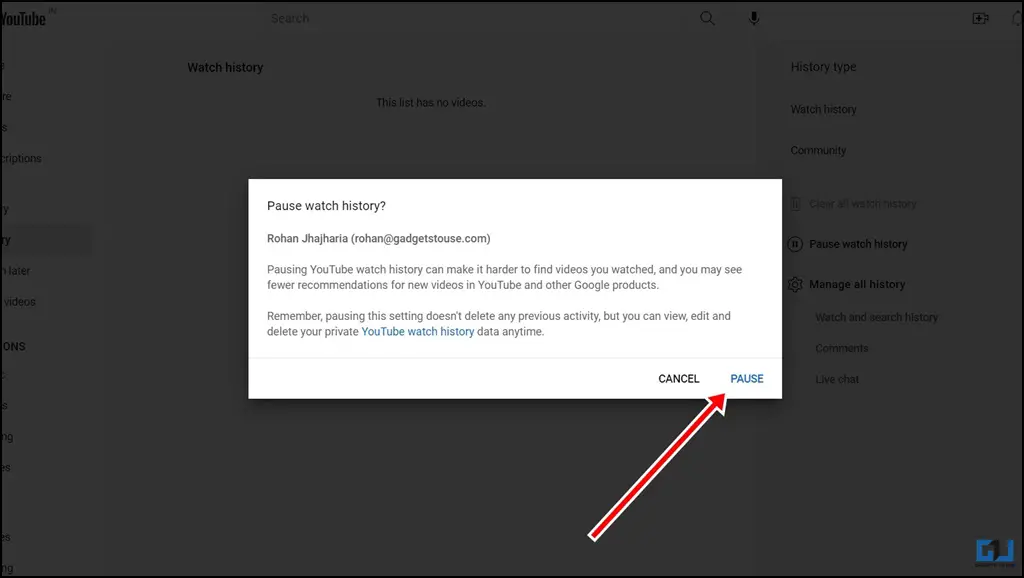This image is a screenshot of a computer displaying a YouTube interface, with the screen slightly grayed out to highlight a central pop-up message. The main focus is a white, horizontal rectangle centered on the screen. Within the rectangle, a message in black text reads: "Pause watch history?" followed by the name "Rohan Johariya" and an email or web address. The message continues to explain that pausing YouTube watch history may make it harder to find previously watched videos and result in fewer video recommendations on YouTube and other Google products. It also clarifies that pausing the setting does not delete any previous activity, and users can view, edit, or delete their YouTube watch history data anytime.

In the bottom right corner of the pop-up, there are two buttons: a black "Cancel" button and a blue "Pause" button. A prominent red arrow originates from the bottom center of the image, pointing directly at the blue "Pause" button, suggesting an emphasis on this action.

The background, although grayed out, is still partially visible. The YouTube logo is located in the upper-left corner, while the top-center text reads, "This list has no videos." To the left of this text, there is a label that says "Watch history." On the right side of the screen, a list of options is visible, including "History type," "Watch history," "Community," "Pause watch history," and "Manage all history." This context indicates the image is related to YouTube's watch history settings and the options available for managing video history.